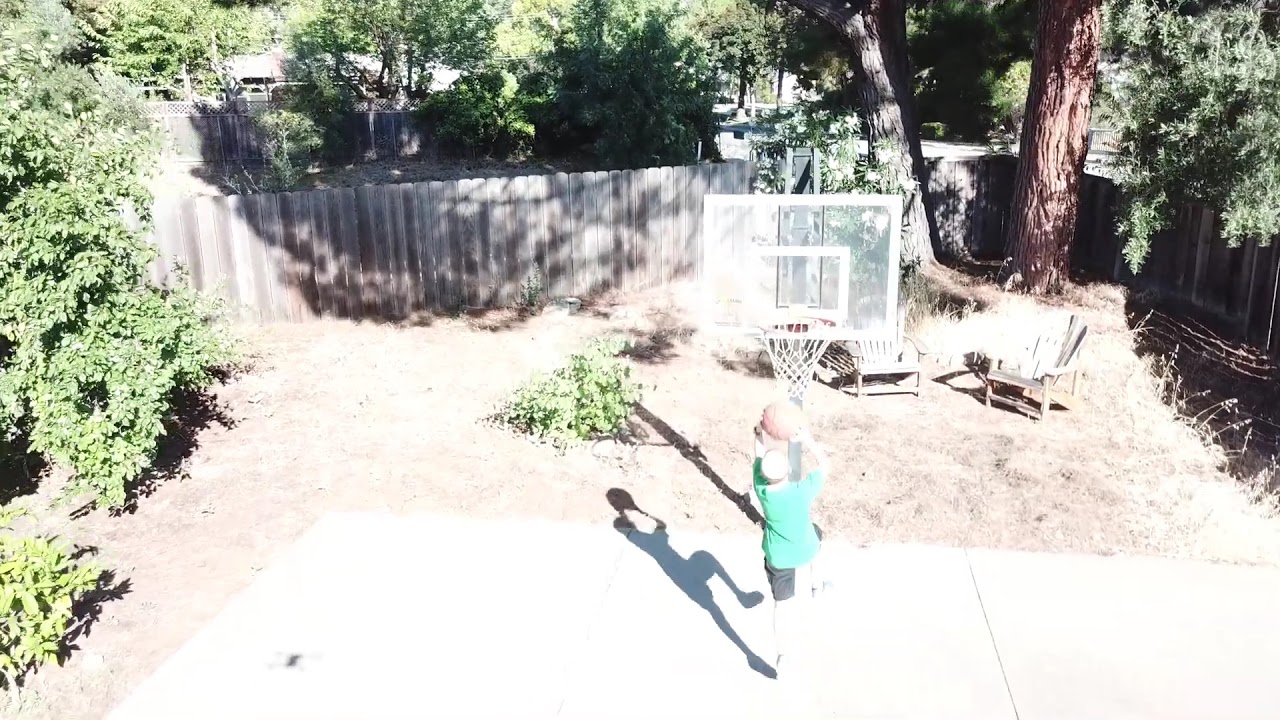In this vibrant and sunlit backyard scene, a young boy, wearing a green shirt and black shorts, is captured mid-action as he attempts to make a basket. With the faded orange basketball raised above his head and his hands poised mid-shot, the boy is positioned toward the bottom center of the image. Directly above him, the basketball hoop features a translucent backboard, possibly made of glass or plastic, with a white net. The concrete slab serving as the basketball court sits beneath him, with his shadow cast towards the left.

Surrounding this main action, the backyard is enclosed by a brown wooden fence, adorned with shadows cast by the tall green trees with robust brown trunks that border the left and right sides of the scene. A couple of wooden chairs are placed against the backdrop of trees and fence, signifying a casual outdoor setup. Adding to the atmosphere, patches of dead brown grass mingle with spots of green, enhancing the naturalistic feel of the setting. The overall brightness and the various shades of green, brown, and gray captured bring a lively and dynamic essence to the image as it highlights a moment of playful activity.